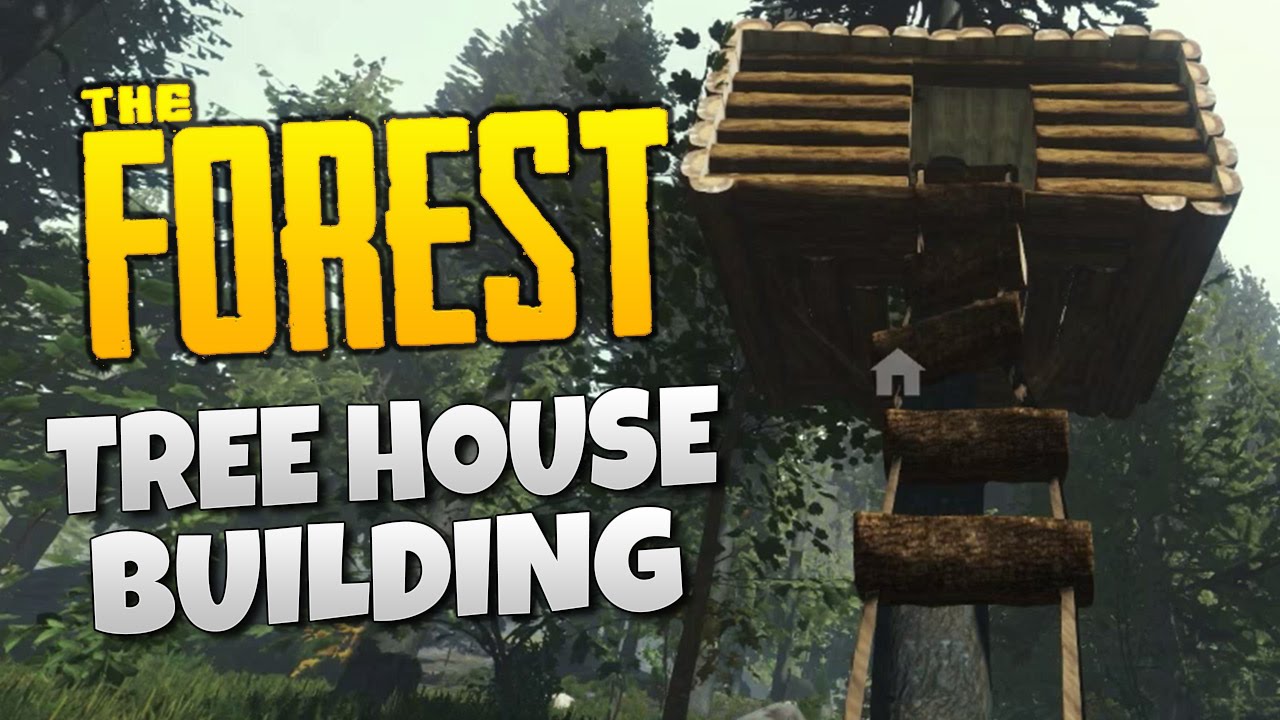The image appears to be a computer-generated or video game screenshot depicting a rustic treehouse constructed from rough logs, reminiscent of Lincoln logs. This treehouse is built around a prominent tree trunk, with a primitive ladder made of logs and ropes leading up to it. The scene is set in a densely forested area with numerous trees partially obscuring a bright sky above. The foreground and background are filled with shades of green from the foliage. To the left of the treehouse, bold block lettering in vibrant yellow and orange spells out "The Forest," followed by "Treehouse Building" in silver text with a black outline. A small home icon is displayed on the wooden steps of the ladder, suggesting a home or safe point within the game. This detailed and immersive depiction suggests a thumbnail for a YouTube video or a website related to the game.